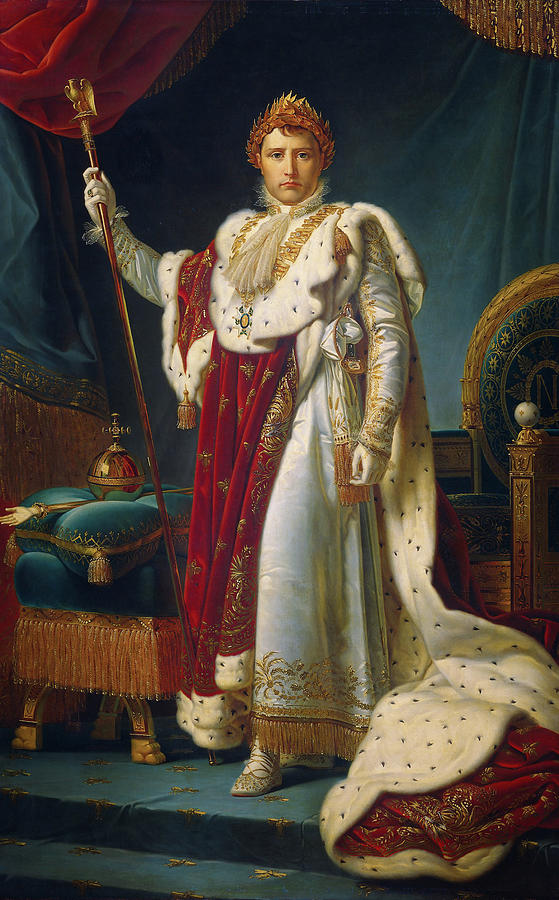The image portrays Emperor Napoleon in his coronation robe, standing in a detailed and ornate setting. He is dressed in an elaborate, velvety gown primarily white, adorned with red and gold tassels hanging from the bottom, and wears white gloves. Draped across his shoulders is a luxurious cape, white with a black pattern on one side and red with gold trim on the other, trailing on the floor and curling behind him. His head is crowned with a golden, leaf-like circlet, and his intense blue eyes are fixed on the viewer. In his right hand, he holds a tall staff topped with an eagle. To his side, there stands a chair characterized by intricate gold legs and a tall, segmented green cushion. Atop the chair sits a metallic, gold container crowned with a cross. The background is rich with diverse hues, featuring blue fabric draped across the walls and a hint of red cloth in the upper left corner. The room is brightly lit, with the detailed decorations and colors vividly captured. There are no borders, text, or any other figures in the image.